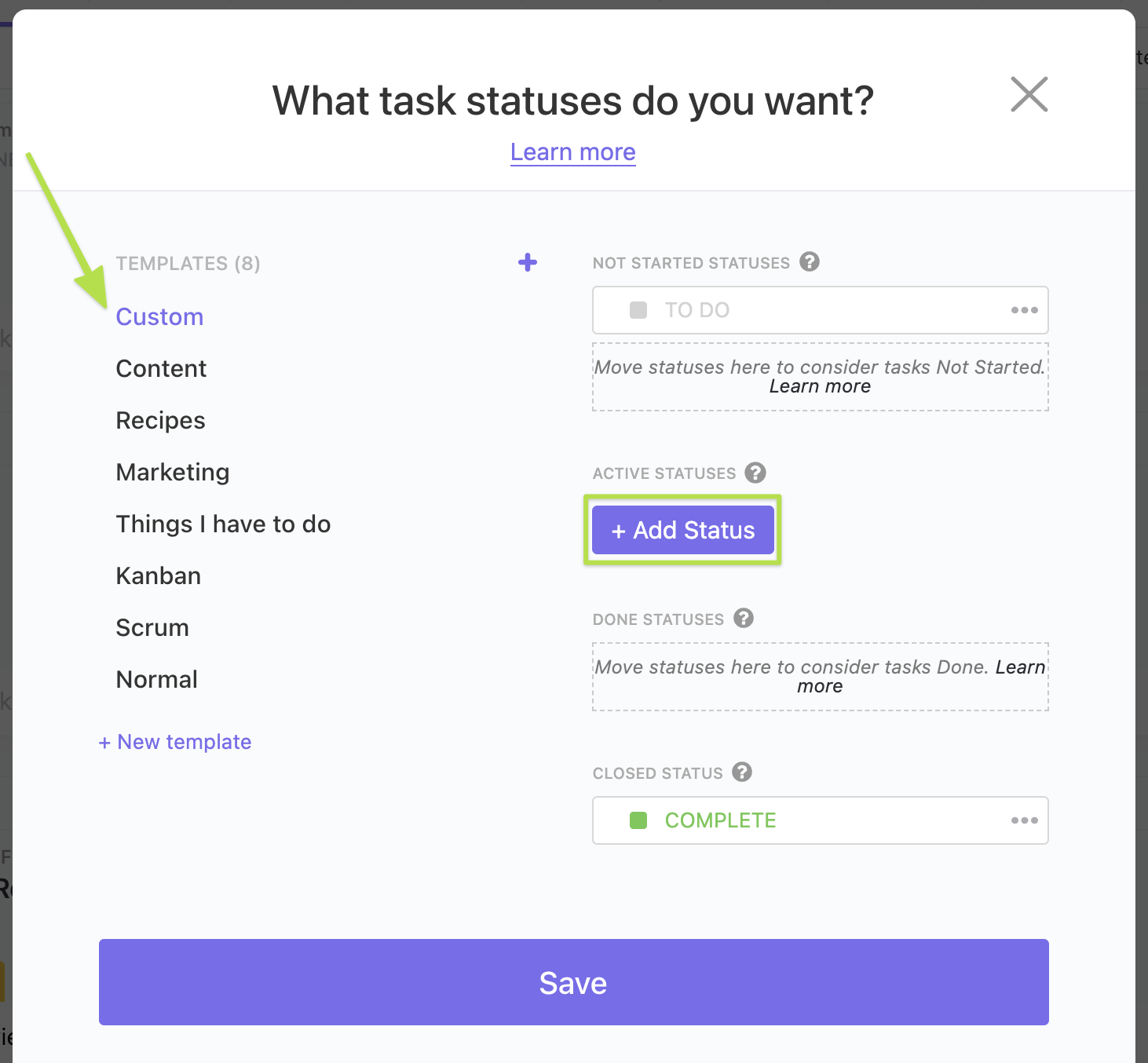The image features a complex interface, segmented into distinct sections with various texts, icons, and colors providing information and navigation options.

At the top, the background is gray, transitioning to black at the uppermost part. Prominently, there's text in white reading, "What would a capital W test statutes do you want?" Below this text, "Learn More" is underlined in purple.

Stretching horizontally across the interface is a bar labeled in gray as "Templates" with an adjoining numeral "8". Adjacent to this, a purple plus sign appears with the inscription "Custom" beneath it. There's a green arrow pointing to this section.

Further below, black text lists categories such as "Content and Recipes" and "Marketing," followed by task indicators like "K and B" and "Scrum," which are presumably project or task tags. One icon reads "New Template" near a plus sign.

To the right, in gray, there's a section titled "Not Started Statutes" with a "To Do" label. Beneath this, black text indicates, "Moustache is here to consider a test," followed by another "Not Started" status and "No More" listed as accurate statuses.

There is also a purple rectangle with an embedded white plus sign, labeled "Has that status," and outlined by a green border. Below this, another gray section denotes "Done Statutes," with an adjoining black text, "Move Statues Statuses here to consider test done," and right after, another "No More."

Towards the bottom, in all capital letters, "CLOSE STATUS" appears next to a gray circle containing a white question mark. Underneath, a white box states "COMPLETE" in green, framed by a green square.

Finally, at the bottom is a prominent purple rectangle, within which "SAVE" is written in white capital letters.